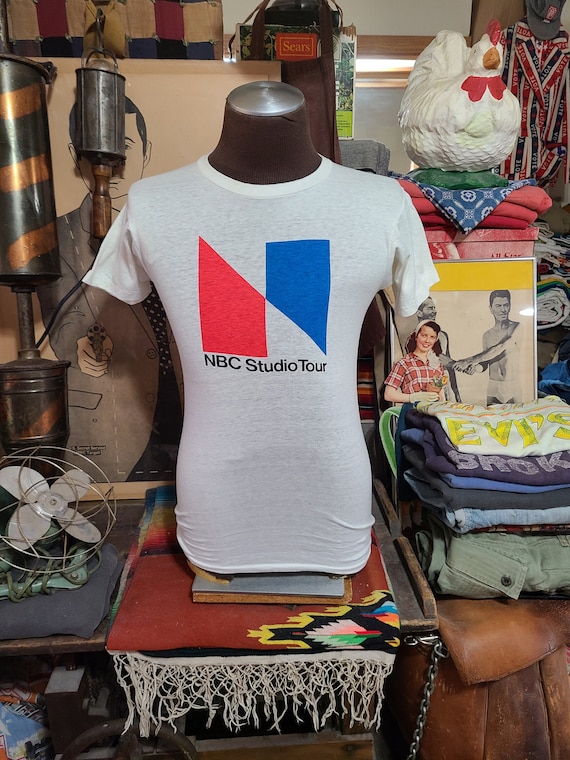This photograph, likely taken in an antique or thrift store, showcases a cluttered interior filled with various intriguing items. At the center of the image is a headless, dark gray mannequin displaying a white t-shirt. The t-shirt features a graphic with red and blue irregular quadrilaterals forming an irregular square, bearing the words "NBC Studio Tour" beneath it. The mannequin is set on a book placed on a carpet, adding to the eclectic arrangement. To the left of the mannequin, a vintage metal fan rests on a brown wooden table. There's also a Southwestern-style blanket with white fringe, folded neatly on the table. To the right, a pile of folded clothes sits atop a brown leather purse with a metal strap. Above this pile, an old photograph of Ronald Reagan is visible, and in the top right corner, a white and red ceramic or plastic hen is perched. Additionally, there is a green and gold trophy-like structure on the left side and a poster depicting a man holding a gun aimed at the viewer. The overall scene is rich with a variety of textures and historical references, evoking a sense of nostalgia amidst the aged and varied objects.